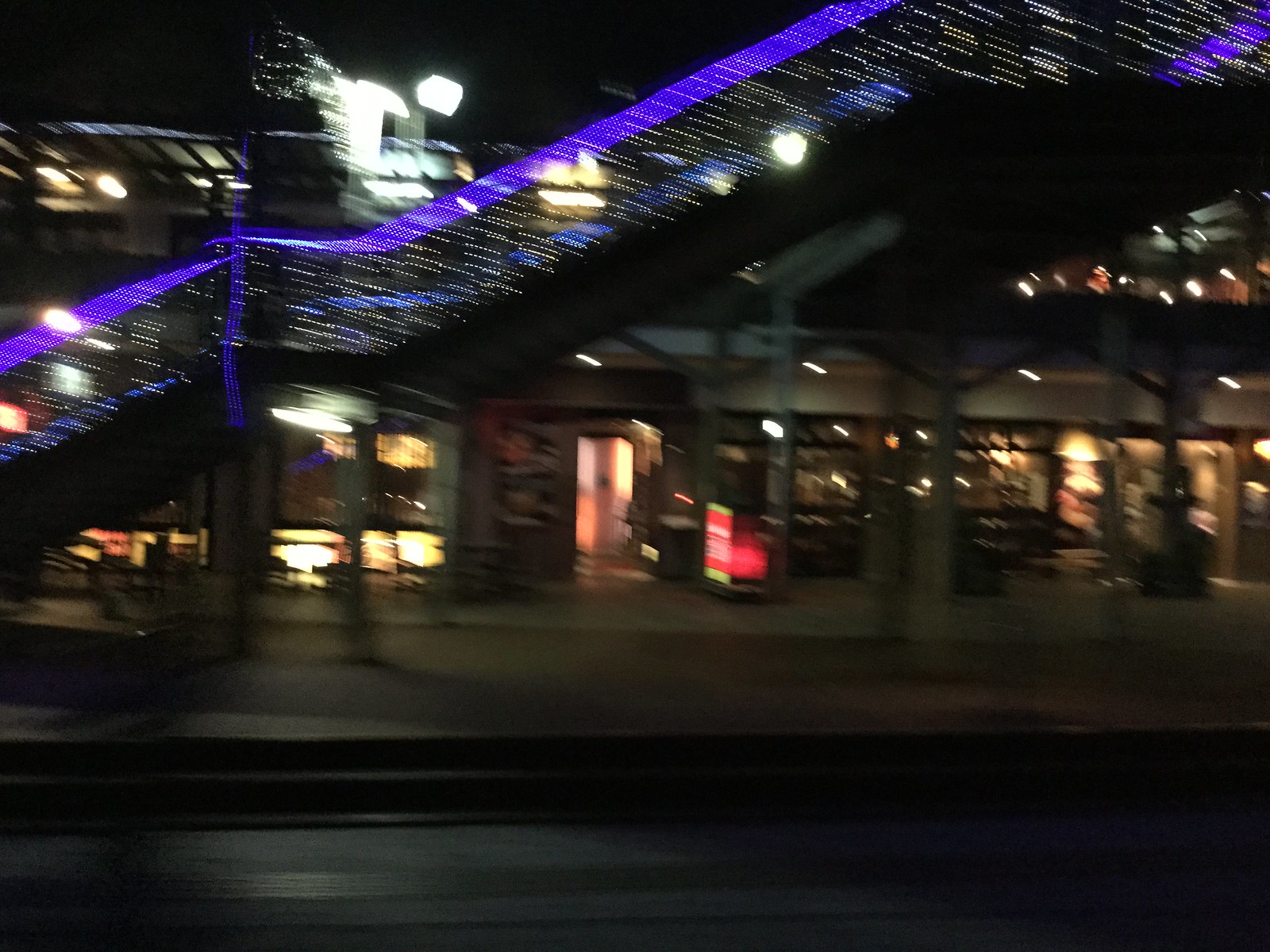This nighttime photograph, though slightly blurry, captures an outdoor scene dominated by a dark street that transitions into a dark gray sidewalk in the foreground. Illuminated buildings with bright storefronts and doorways populate the background, their lights providing a stark contrast to the night. Awnings are visible above the stores, adding a layer of architectural detail to the scene. On the left side of the image, a hazy blue structure, potentially a roof, appears streaky and indistinct, with lights adding a mysterious glow to this part of the composition.